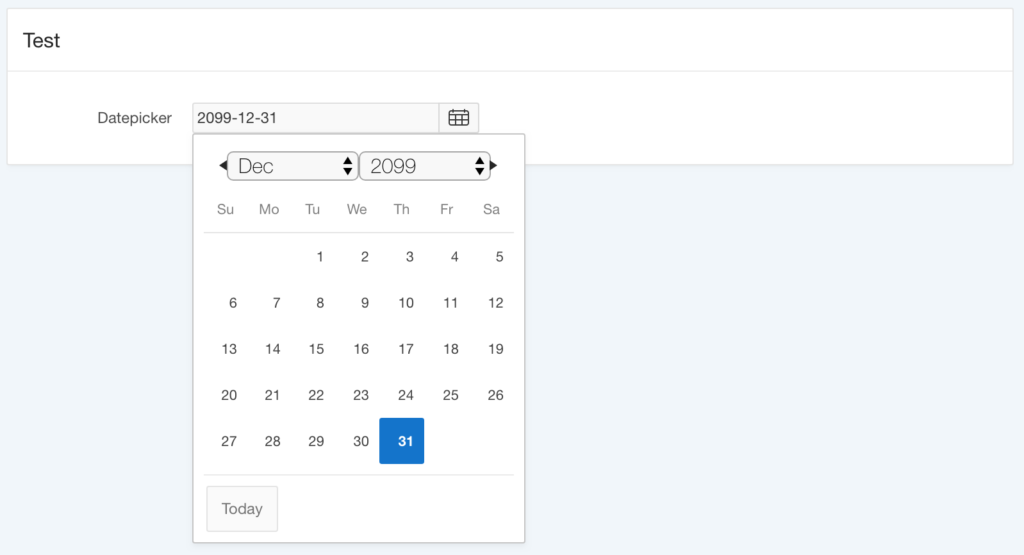The image is in landscape format, with a white banner stretching across the top from left to right. The banner is divided by a light grey horizontal line. In the top left corner of the banner, the word "Test" is displayed in bold black lettering. Below the dividing line, the banner reads "Date Picker," beneath which there is an interactive text box.

The text box currently shows the date "2099/12/31," indicating the 31st of December, 2099. To the far right of this text box, there is a calendar icon, indicating that the calendar is expandable. Indeed, the calendar is expanded in this image, showing all 31 days of December 2099. The days of the week are abbreviated at the top of the calendar as follows: S-U-M-O-T-U-W-E-T-H-F-R-S-A, corresponding to Sunday, Monday, Tuesday, Wednesday, Thursday, Friday, and Saturday.

Within the calendar grid, the number "31" is prominently highlighted in blue, indicating that the selected date, December 31, 2099, falls on a Thursday. Below the calendar, there is another dividing line, and beneath that, a grey box labeled "Today."